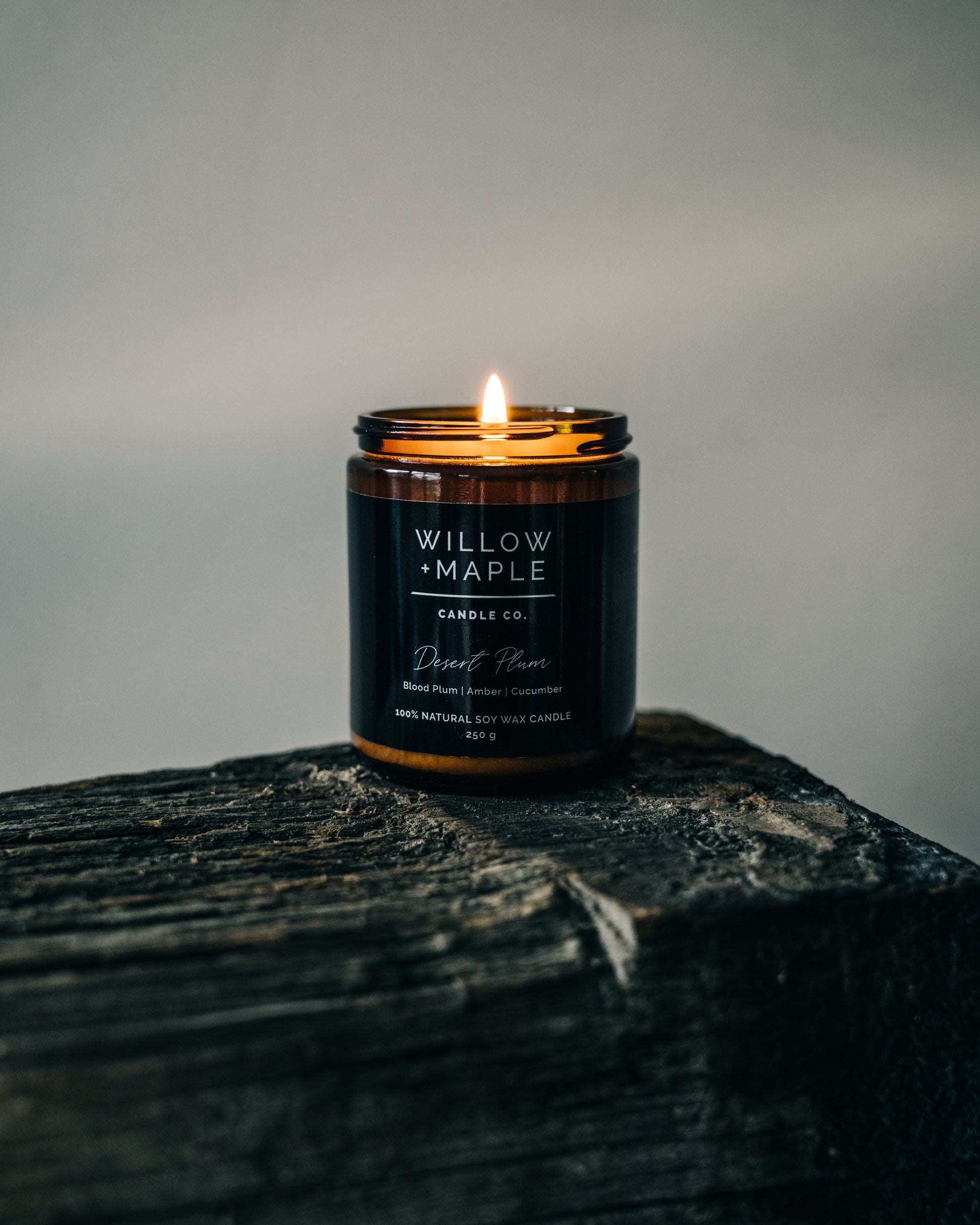This detailed photograph features a stylish and rustic amber-colored glass candle with a lit yellowish-white flame, exuding a warm, inviting glow. The candle bears a sleek black label with white text, reading "Willow and Maple" in bold capital letters, followed by a white line and the words "Candle Company." Below, the scent name "Desert Plum" is elegantly scripted, followed by the fragrance notes "Blood Plum, Amber, Cucumber" in standard print. The label also highlights "100% Natural Soy Wax Candle, 250 grams" in all capital letters.

The candle is positioned on a large, weathered wooden block with a dark, almost charred appearance, contributing to its masculine and rustic feel. The background remains understated with a blurry gray tone, allowing the candle's warm, amber hue and the rustic wooden surface to take center stage in this modern, stylish product image.